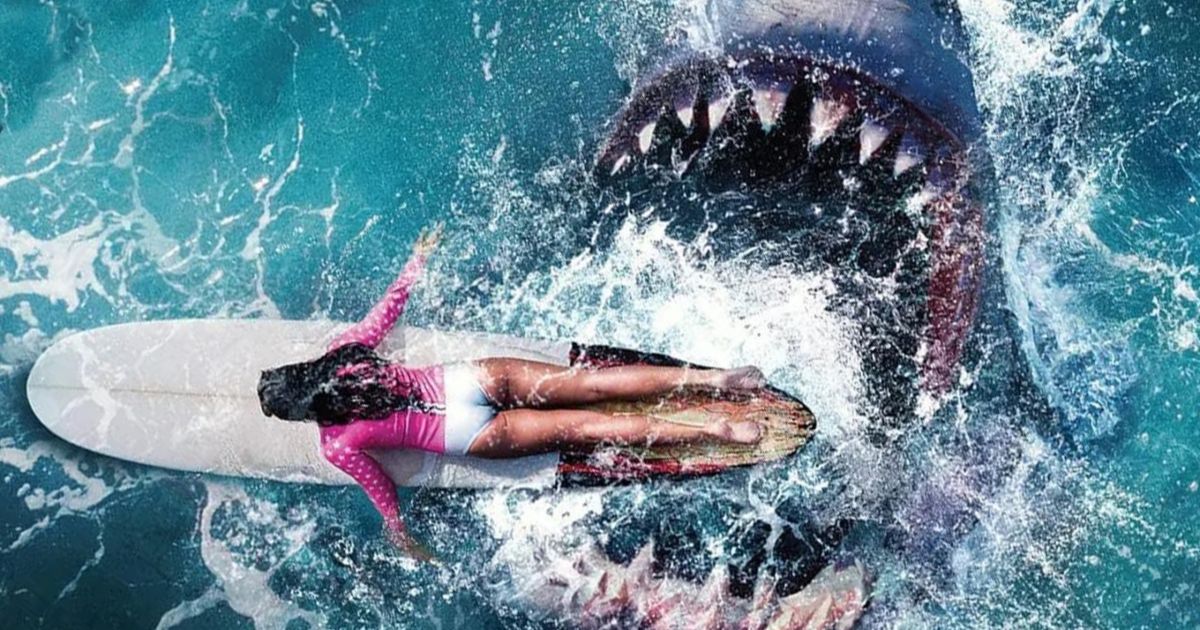In this dramatic scene, a woman is lying on her stomach on a white surfboard with a distinctive line running down the middle, floating amidst the teal, bubble-filled waters. She has long black hair cascading down her back and is dressed in a pink long-sleeved top adorned with white dots, paired with tight-fitting light blue bottoms that cling closely to her form. Her bronze-skinned legs are extended behind her, with her hands dipping into the water as though she's paddling. Unbeknownst to her, a large shark with menacing teeth — white on both its upper and lower jaws — is emerging from the water, its mouth wide open, directly below her feet. The shark, mostly obscured by the frothy, white splash of water, reveals its blue-gray skin beneath the tumultuous waves, poised to strike. The scene is a dire juxtaposition of serene paddling and imminent peril, highlighted by the turbulent splash of the shark's dramatic entry.